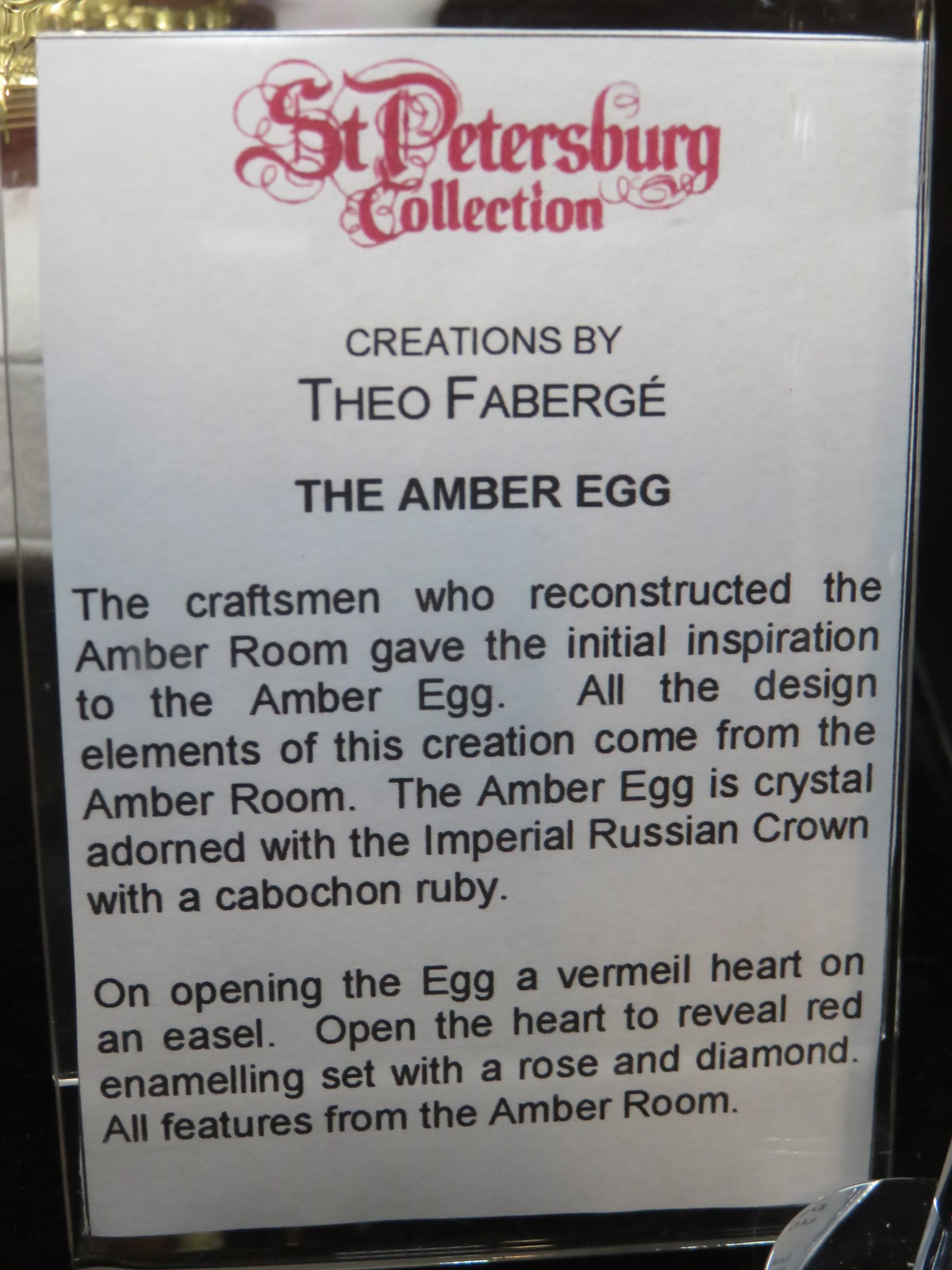The image displays a laminated informational placard from the St. Petersburg Collection. At the top, in ornate red calligraphy with flourishing details, it reads "St. Petersburg Collection." Below that, in black capital letters, it states "Creations by," followed by "Theo Fabergé" and then "The Amber Egg" in bold. The text goes on to describe that the craftsman who reconstructed the Amber Room provided the initial inspiration for the Amber Egg and that all design elements originate from the Amber Room. The Amber Egg is made of crystal, adorned with the Imperial Russian crown, and features a cabochon ruby. Upon opening the egg, it reveals a vermilion heart on an easel; when the heart is opened, it unveils red enameling set with a rose and diamond, all elements reflective of the Amber Room's features. The placard is encased in glass, reflecting a metallic object in front of it, which appears silver or chrome. The bottom of the placard includes a web address for the Global Oneness Project.